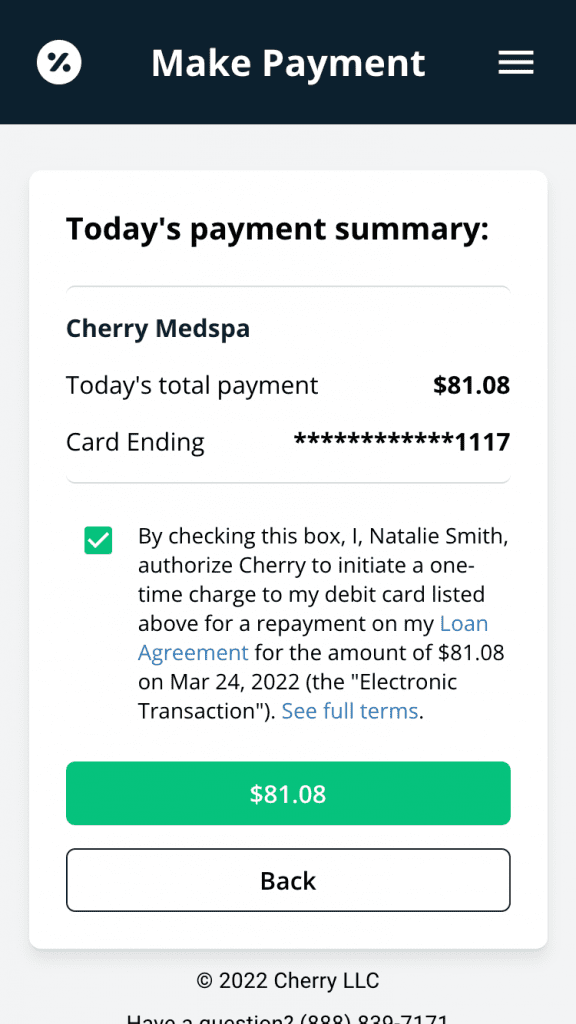The image displays an online payment portal, likely a pop-up window, for Cherry Med Spa. At the top of the portal is a black header with the text "Make Payments" centered. To the right of the header, there are three horizontal lines stacked, indicating a drop-down menu.

The main content of the portal features a white background. Below the header, the text "Today's Payment Summary:" is displayed, followed by a list that includes:

- "Cherry Med Spa"
- "Today's Total Payment: $8108"
- "Card Ending: 1117"

There is also a detailed authorization statement which reads: "By checking this box, I, Natalie Smith, authorize Cherry to initiate a one-time charge to my debit card listed above for repayment on my loan agreement for the amount of $8108 on March 24, 2022 (the electronic transaction). See full terms." The phrases "loan agreement" and "see full terms" are hyperlinked and colored blue.

A checkbox with a green background and a white checkmark is situated next to the authorization text. Below that, a green button displays the amount "$8108" in white text. Directly beneath this is a white button, outlined in black, with the word "Back" in black text.

At the bottom of the portal, the text "Copyright 2022, Cherry LLC" is visible. Part of the text below seems to be obscured, but it likely reads "Have a Question" followed by a phone number.

The color scheme used includes black, white, gray, blue, and green.